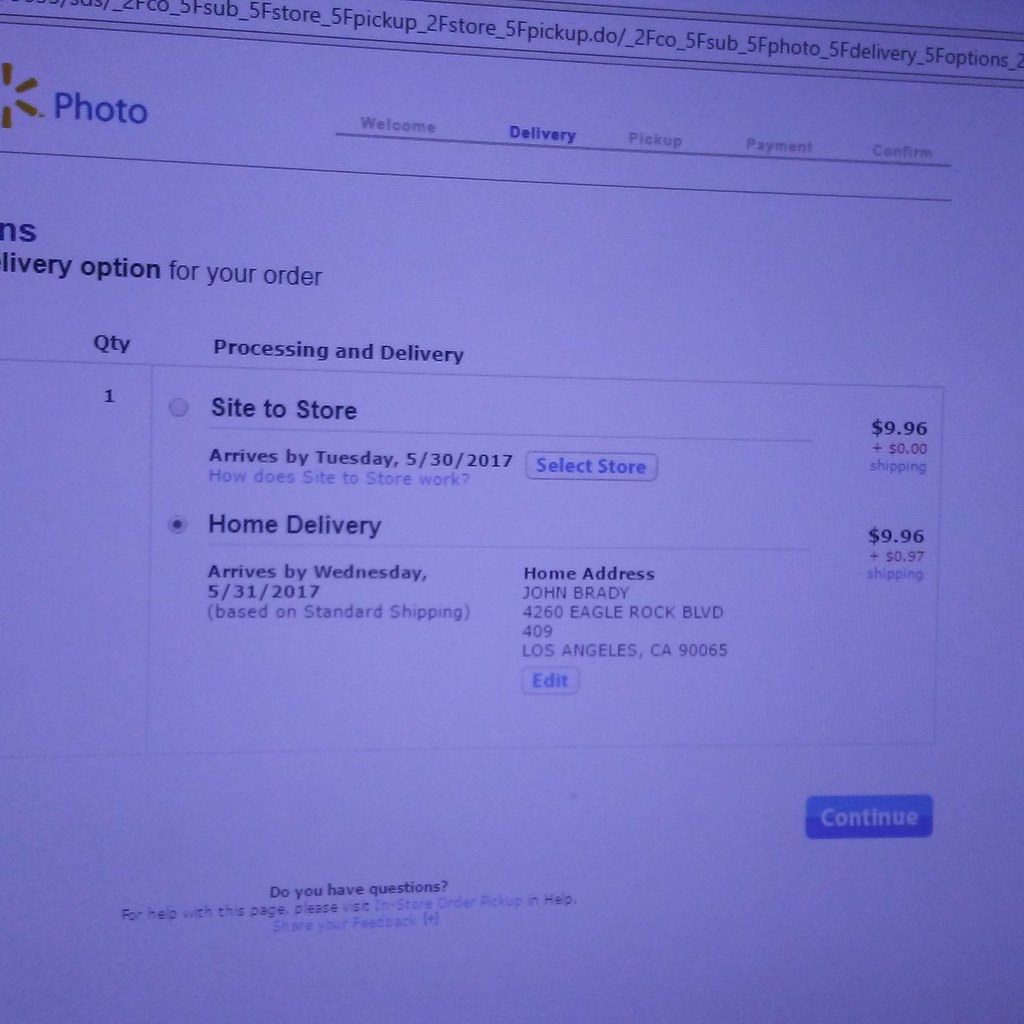A photograph captures a computer screen displaying the Walmart website with a blue tint, likely due to the environmental lighting. The upper left corner of the screen shows a partial Walmart logo, accompanied by the word "Photo," indicating that the website's photo service is being used. The user has selected to have photos delivered, and the screen details the order specifics: a single photo (Quantity: 1) is being purchased with home delivery selected. The anticipated delivery date is Wednesday, May 31, 2017, based on standard shipping. The shipping address listed is John Brady, 4260 Eagle Rock Boulevard, Apt. 409, Los Angeles, CA 90065. The total cost of the order is $9.96 plus an additional $0.97 for shipping, making the screen a comprehensive snapshot of a transaction in progress.